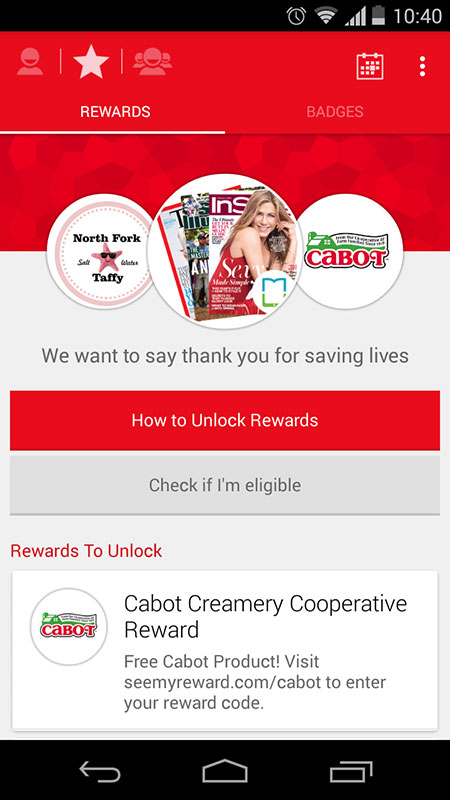The screenshot displays a smartphone interface with a black border at the top. In the upper right corner, "10:40" is written in white font, alongside icons indicating the battery is approximately 25% charged, a Wi-Fi signal, and an alarm clock. Below this, the header features a red background with three circles. 

The right circle displays the Cabot logo, a cheese company logo in red with a green banner at the top. The center of the image showcases a stack of magazines fanned out, with "InStyle" magazine at the forefront, featuring a white woman with long light brown hair in a red strapless dress. The left circle contains the "North Fork Taffy" logo, accompanied by a small cartoon star.

At the bottom, a white strip contains the text "Cabot Creamery Cooperative – Reward: Free Cabot Product," followed by a website address. The Cabot logo appears again to the left of this text.